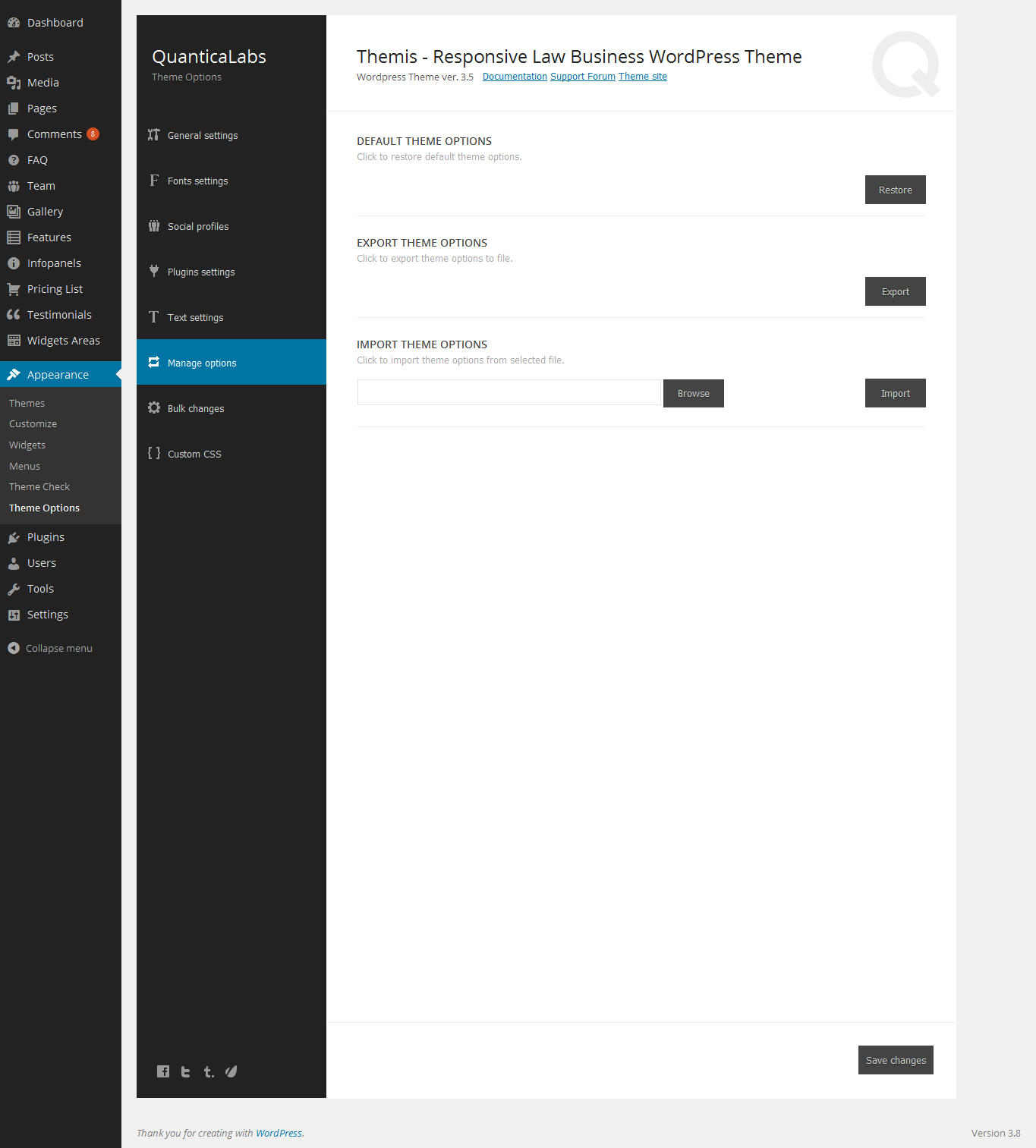This is a screenshot of a website's theme adjustment interface. On the right side of the image, there is a narrow vertical rectangle containing various tabs. The active tab is highlighted with a black background, featuring white text and icons, except for the "Comments" section, which has an orange circle with a white symbol inside it. Directly below is the "Appearance" tab, marked with a blue rectangle and a right-facing arrow that leads to another section labeled "Quantica Labs." This section also lists "Theme Options" in white text against a blue background.

The interface offers detailed controls for theme customization, including options to change the theme, restore the default theme, export the theme, or import theme options. At the bottom of the interface, a "Save Changes" button is prominently displayed, ensuring that users can securely apply their customization choices.